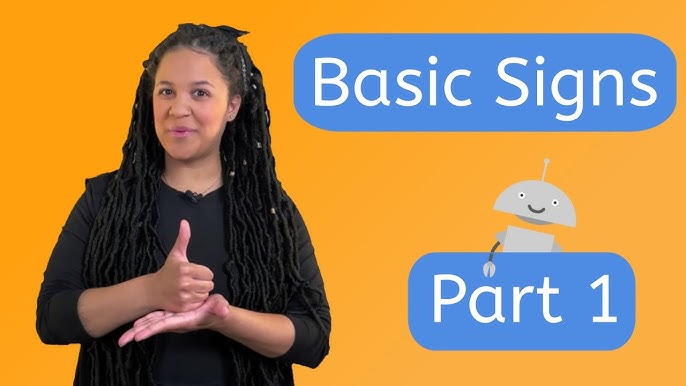The image features an African American woman with long braided hair, positioned on the left side. She appears to be in her 30s and is demonstrating a sign language letter, with her thumb raised. She is dressed in a black quarter-length sleeve shirt. The background behind her is orange. To her right, there is a blue banner with white lettering that reads "Basic Signs." Below this banner, another blue banner states "Part 1," accompanied by a cartoonish gray robot with a cheerful expression, two white eyes, an antenna, and one of its hands draped over the banner.